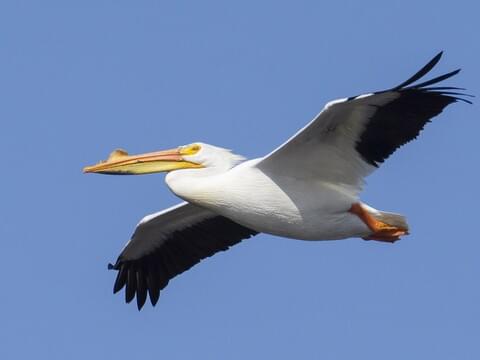The image depicts a large bird, likely a pelican, soaring gracefully in a clear, bright blue sky devoid of clouds. The bird's body is predominantly white, with distinctive black markings on the wings, particularly under the wing and at the tips. Its wings are fully spread, displaying a slight separation of feathers near the ends, suggesting a fluid glide rather than active flapping. The bird features a long beak that is light orange at the top and yellow at the bottom, with a small orange notch approximately a quarter of the way down from the top. Its eyes are surrounded by a yellow ring, adding to its striking appearance. The bird's feet are dark orange, and they dangle slightly as it moves through the air. Despite the bright ambiance of the sky, the sun itself is not visible in the image. The scene captures the bird in mid-flight, as it appears to float effortlessly in the serene atmosphere.